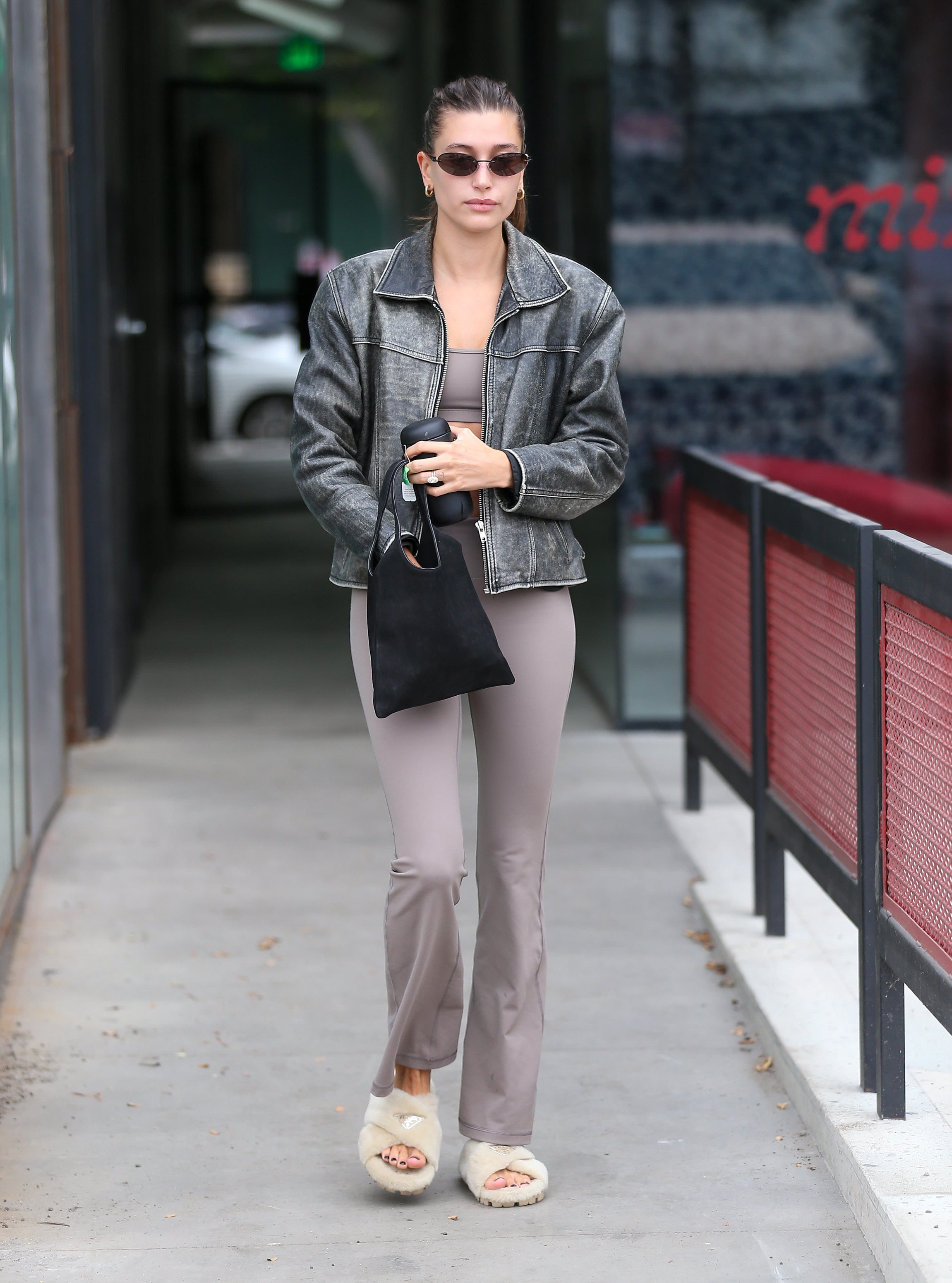The image showcases Haley Baldwin, a young Caucasian woman in her 20s, walking towards the camera along a muted city street. Her dark brown hair is slicked back and tied, falling below her shoulders. She wears oval black wire sunglasses and a faded, worn black leather jacket that reaches her waist. Underneath the jacket, she has on a midriff-baring, mauve-colored sports bra or tank top, matched with form-fitting yoga pants of the same shade that flare into a wide-leg cut below the knee. On her feet, she sports fluffy beige slippers, revealing her toes painted in a striking black color. Haley is clutching a small black purse in her left hand, which also shows her wedding ring, and holding what appears to be a black cell phone in her right hand. The background features a partially visible red bench with brown wood.